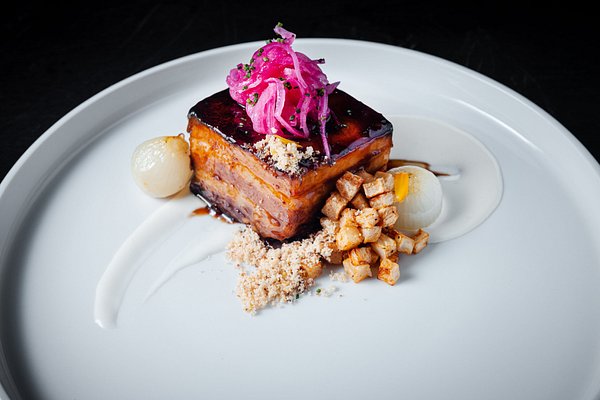This photograph, seemingly taken indoors, showcases a meticulously crafted gourmet dish on a large, pristine white ceramic plate set against a stark black background. The focal point is a square piece of braised and deep-fried pork belly, displaying rich layers of gold, tan, and brown. This main component is topped with a generous heap of shredded, pickled red onions, adding a vibrant pink contrast.

Flanking this centerpiece, on the left side of the plate, rests a notable small white onion, while scattered miniature croutons and small cubes of potatoes decorate the right side. Additionally, a shimmering gold granular substance is sprinkled in front of the pork belly, and a few granules have artistically fallen onto the plate.

The entire arrangement is elevated by a delicate smear of a white cream or sauce, possibly a glaze, which underpins the pork belly and spreads elegantly across the plate, enhancing the visual appeal with its glossy texture. This elaborate presentation, accentuated by careful placement and diverse textures, suggests it is a high-end entrée or appetizer, likely an expensive and exquisite culinary creation.